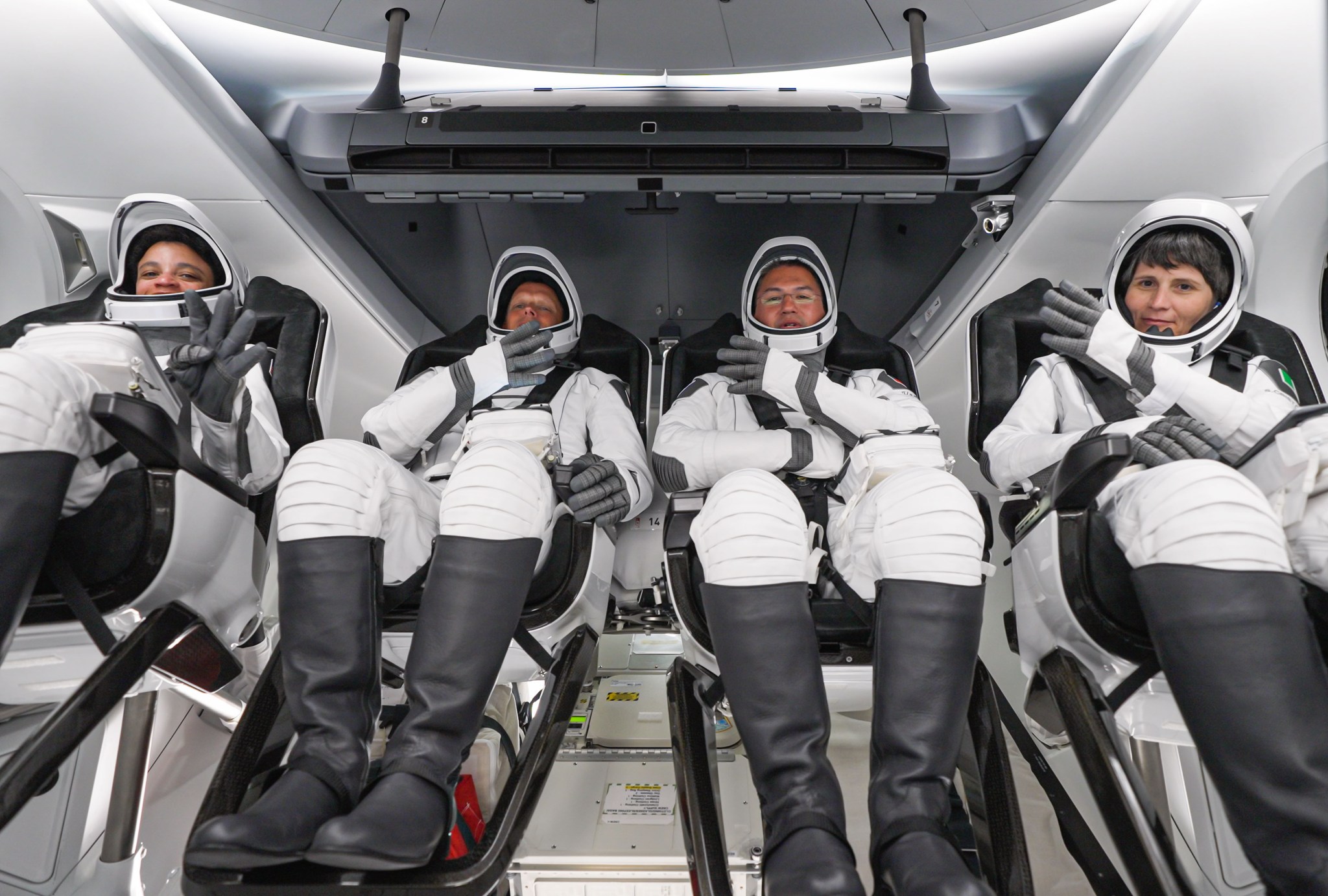In a close-up shot, four astronauts are seated in a sleek, white cockpit or training module, each secured into black backrest chairs with black footrests. They are dressed in matching space suits with black boots, white segmented legs and shirts, and gloves with gray fingers and wrist accents. Their white helmets, featuring open face masks, reveal their faces. 

The astronaut on the far left is a woman with dark brown skin, smiling and holding up four fingers on her left hand. The next astronaut, a white man with his eyes closed, leans back in his seat. The middle-right astronaut, a sunburned white man with raccoon-like white patches around his eyes, rests his left elbow on his knee, also holding up four fingers. The far-right astronaut, a white woman with black hair, rests her left elbow on her knee, her face clearly visible. Behind them, a gray control module descends from above, framed by a triangular opening in the background.